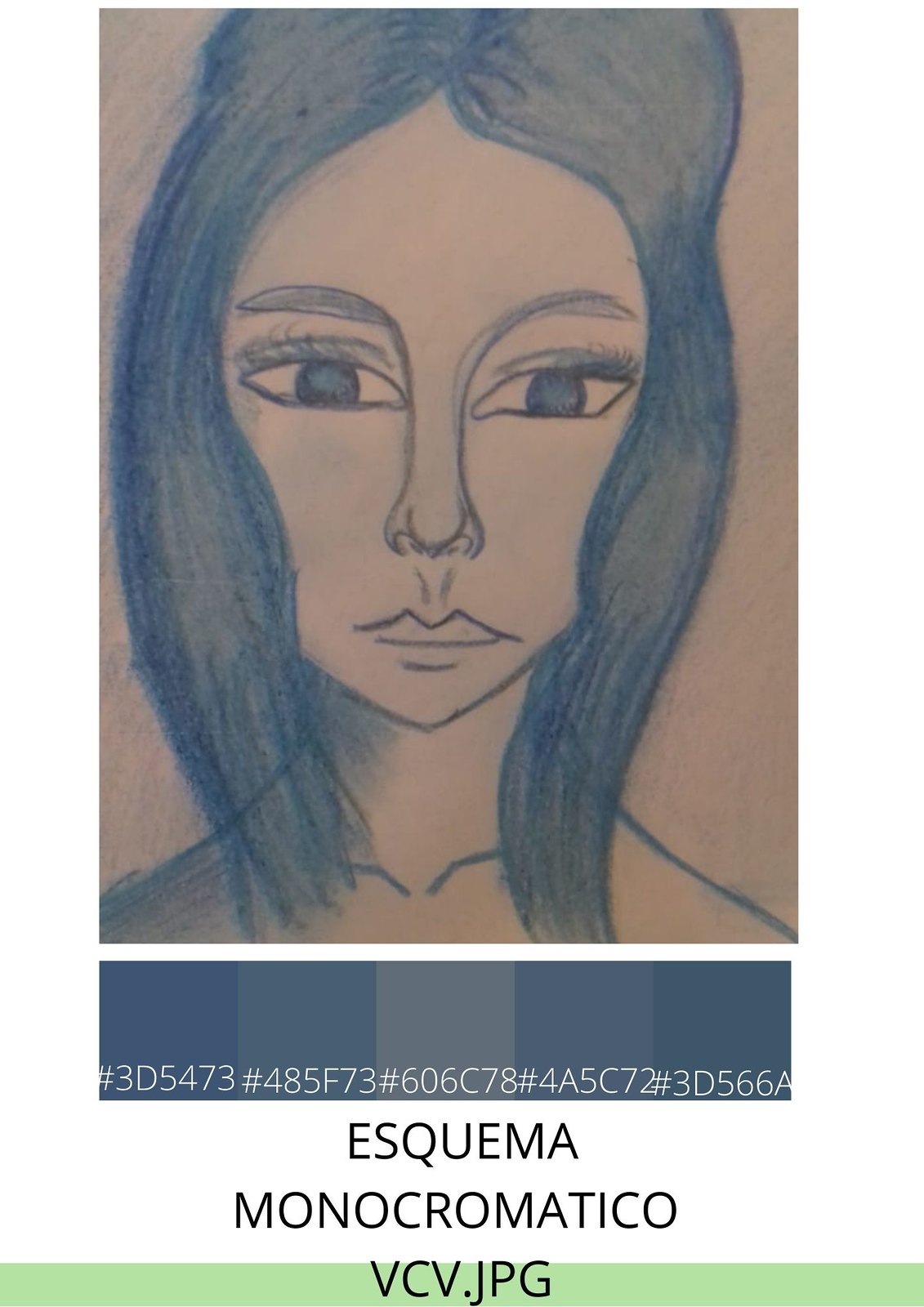The image is predominantly a tall, narrow piece, standing about two and a half times taller than it is wide. The central focus of the image is a pencil or charcoal drawing of a woman. She has large, oval, dark-centered eyes with no visible pupil or iris differentiation, and is facing forward. Her long black hair cascades to her mid-collarbone and features a high bump in the back, reminiscent of Amy Winehouse's hairstyle. The woman's face includes dark eyebrows, a long nose, and an almost triangular mouth, with light sketch lines indicating the contours around her mouth and collarbone.

The background of the drawing is off-white. Beneath the drawing, there is a horizontal transition of five different shades of navy blue. Directly below this gradient, a string of 20 random characters, including letters, numbers, and pound signs, runs across the width of the image. At the very bottom, there is a thin light green rectangle occupying less than 5% of the image's height. Within this bar, written in three lines of black capital letters, is the text "ES-Q-U-M-E-M-A MonochromaticoVCV.jpg," which appears to be the file name. The intricate detailing of the woman's facial features, combined with the underlying color elements and textual components, make this a richly descriptive and complex image.